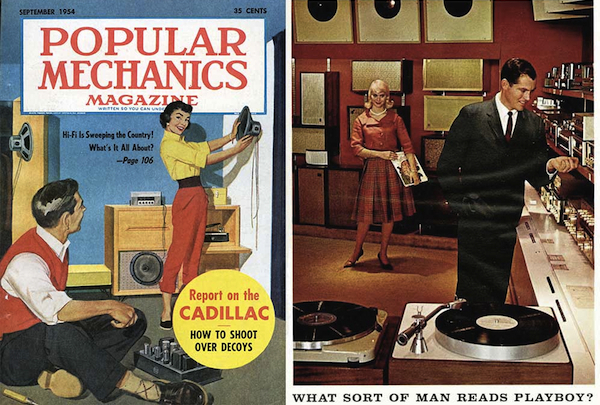The image features a two-paneled design highlighting elements commonly associated with 1950s magazine culture and lifestyle. On the left panel, the cover of a September 1954 issue of Popular Mechanics Magazine is presented. The cover features red text on a white background with a blue border and sells for 35 cents. The prominent headline, "Hi-Fi is sweeping the country, what's it all about? Page 106," is displayed against a blue background. Below, a yellow circle teases articles such as "Report on the Cadillac" and "How to shoot over decoys." The illustration shows a woman with short hair, smiling as she places a speaker on a blue wall. She is dressed in a yellow blouse, red pants, black shoes, and a black belt. On the floor, a man in a light collared shirt, red vest, and black pants works on a radio with various tubes around him.

The right panel contains a retro scene, hinting at a different magazine's exposé titled, "What Sort of Man Reads Playboy?" A man in a black suit with a white shirt and thin tie adjusts the controls of an elaborate stereo system that occupies the entire right wall. Beside him stands a woman in a knee-length red dress with a pearl necklace, holding a record. The room's background features multiple wall-mounted speakers, with dominant red and orange hues, reflecting the stylish ambiance of the time.